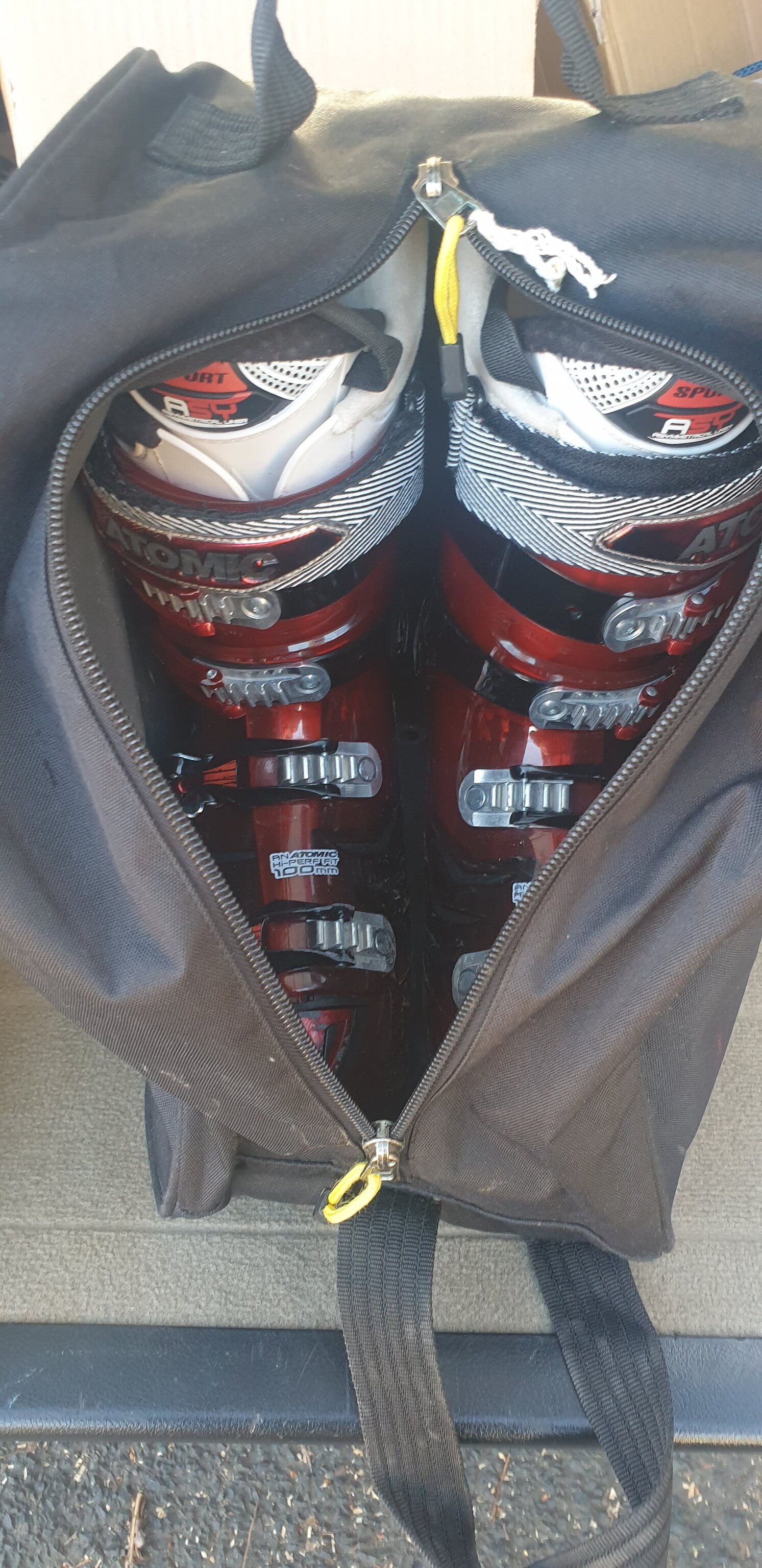This image showcases a pair of rigid, deep-red ski boots with distinctive black stripes and white cuffs peeking out from within a partially unzipped, black duffel bag. The zippers of the bag are silver, each adorned with a small yellow circular object. The duffel bag, positioned vertically, reveals its contents through an open zippered closure that creates a heart-shaped opening. The boots, detailed with silver buckles and transparent white strappings, exhibit a robust design typically used for ski bindings. The scene is set against a concrete floor with a black border and the boot’s branding, “Atomic” in bright, almost metallic red, is distinctly visible—a key feature echoed on both pairs of the boots. Additionally, the bag features a small handle strap at the top and a larger shoulder strap towards the bottom, framed predominantly within the photograph.